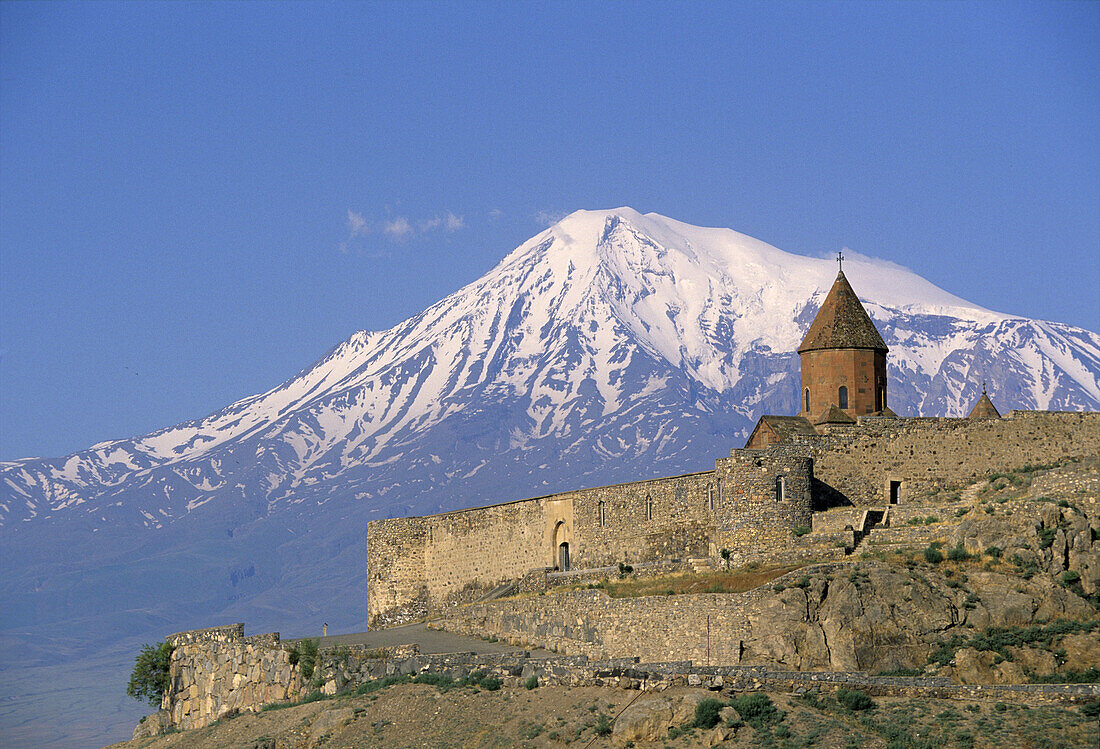A majestic castle, constructed from rich brown bricks, stands proudly in the foreground, slightly to the right, against a breathtaking backdrop of snow-capped mountains. The castle's prominent turret, capped with a matching brown roof, adds a touch of medieval charm to the scene. Above, the sky stretches out in a brilliant, uninterrupted blue, seamlessly blending with the hues at the base of the mountain range, creating a truly remarkable vista. The terrain surrounding the castle is rugged and rocky, interspersed with a few green shrubs that cling tenaciously to the uneven ground, adding a touch of life to the austere landscape.